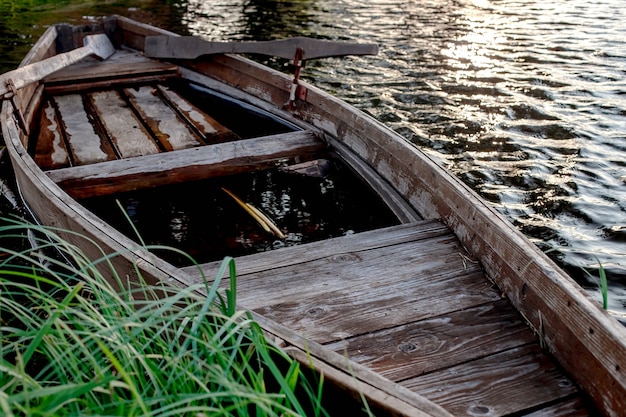A detailed daytime image depicts an old, weathered wooden boat positioned near the shore of a body of water. The boat, faded from dark brown to a worn, almost whitish hue, exhibits signs of age and neglect, with patches of missing wood and some areas partially submerged in water. Inside the boat lie wooden paddles, and there is evidence of water pooling at the bottom, indicating its abandoned state. The body of water, visible in the upper right corner of the image, features gentle ripples and a shimmering reflection of sunlight, casting an orange-ish hue across the surface. The left bottom corner of the image shows a patch of green grass peeking into the scene, adding a touch of life to the otherwise somber setting.